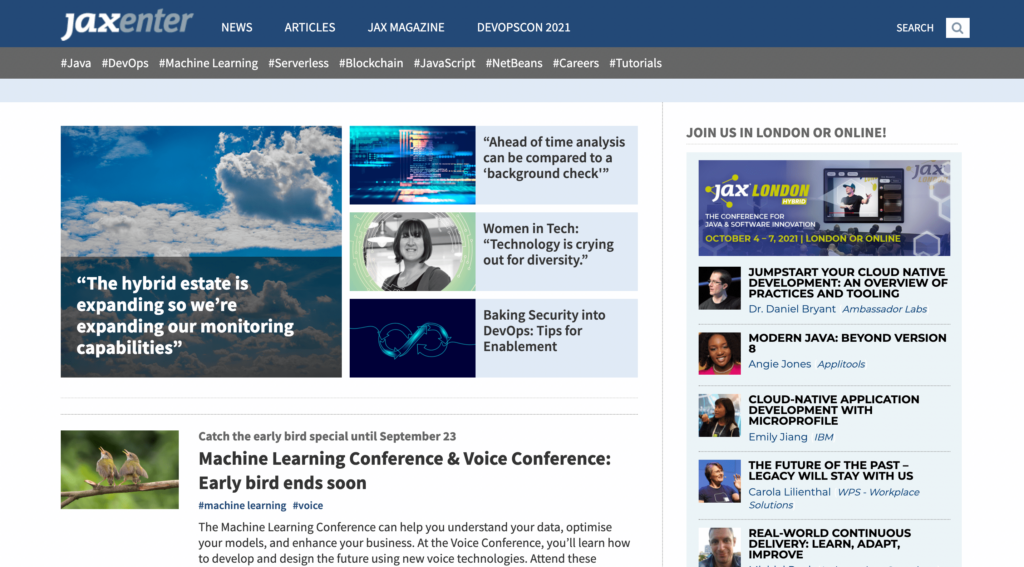Here is a refined and descriptive caption for the given image:

---

The screenshot captures a webpage from the JAXenter website. At the top, there is a prominent navigation bar, with the upper two-thirds in cornflower blue and the lower third in gray. On the left-hand corner of this bar, the website's name "JAXenter" is displayed in white and gray text. The menu options include "Menu Selection," "News," "Articles," "JAXX Magazine," "DevOpsCon 2021," and two search icons.

The gray portion of the bar features several hashtags: "Java," "DevOps," "Machine Learning," "Serverless," "Blockchain," "JavaScript," "NetBeans," "Careers," and "Tutorials." Below this bar, a scenic photo of a countryside with a clear blue sky spans the width of the page.

Adjacent to the photo, there are various sections with headlines like "The hybrid state is expanding, so we're expanding our monitoring capabilities," and "Ahead-of-time analysis can be compared to a background check." Additional snippets showcase content on topics such as "Women in Tech," discussing the need for diversity in technology, and an illustration resembling a DNA strand linked to "Banking Security Info," "DevOps," and "Tips for Enablement."

Further down, an article highlights an "Early Bird Special" for the Machine Learning Conference and Voice Conference, running until September 23rd. It explains that these conferences aim to help attendees understand data, optimize models, and enhance business practices. The Voice Conference focuses on the future of voice technology development and design.

To the right, an advertisement promotes a conference titled "Join us in London or online, JAX London," with various menus providing additional details about the conference offerings.

---

This caption provides a comprehensive description of the webpage contents and its layout, ensuring clarity and detail.